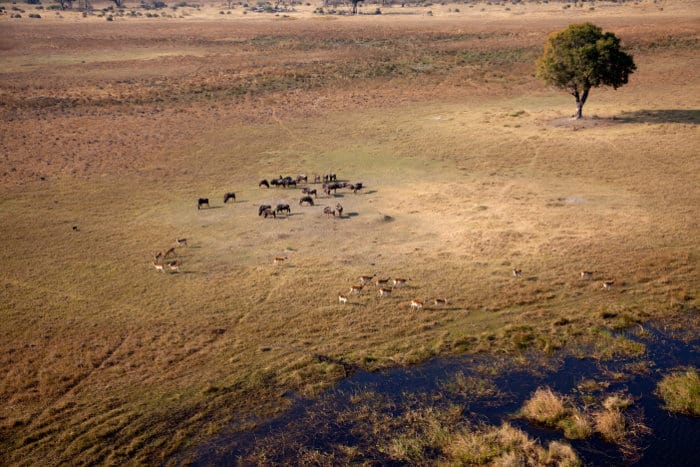This aerial photograph captures a sweeping view of a Serengeti-like landscape predominantly in shades of tan and brown, interspersed with patches of green foliage. The composition is defined by a central, worn brown circular area, heavily trodden by animals, which extends into slightly darker plains. In the immediate foreground, there's a pond adorned with ferns. Scattered across the central clearing are three distinct herds of grazing animals, possibly deer, antelope, elk, or gazelles, forming a triangular arrangement: a darker brown herd at the top, and a lighter brown herd at the bottom. The lone green tree with a Y-shaped fork in its trunk stands prominently in the upper right corner, casting a shadow to the right. The vantage point of the photograph offers no horizon line, emphasizing the vast expanse and the intricate details of the ground below, including the bare patches where the animals have overgrazed.